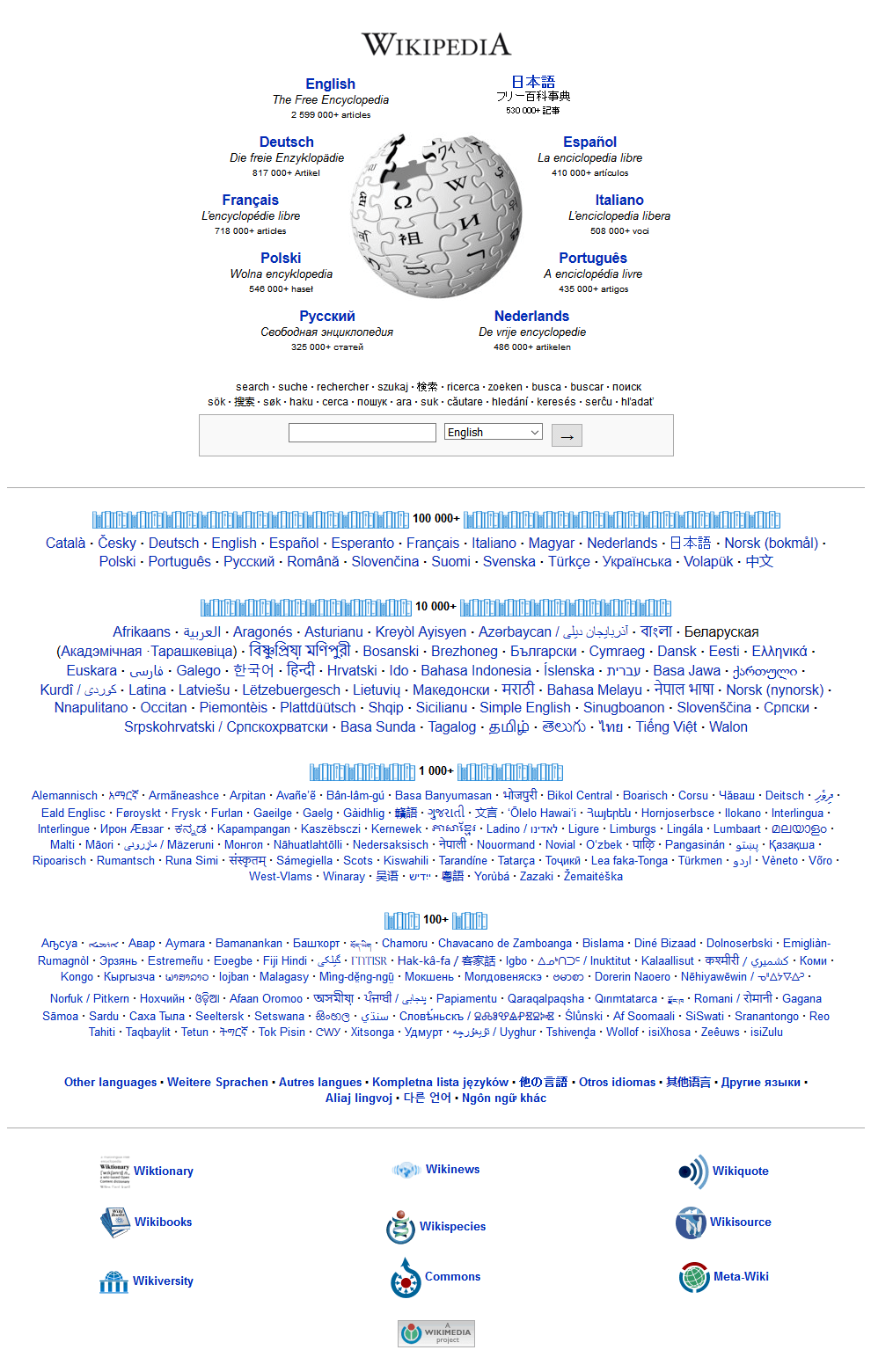This image is a detailed screenshot of Wikipedia’s homepage. At the very top, the word "Wikipedia" is prominently displayed in bold black letters. Directly beneath this title is a distinctive globe, comprised of interconnected puzzle pieces, symbolizing the collaborative nature of the platform. Surrounding the globe are inscriptions in various languages, including English, Chinese, Español, Italiano, Português, Nederlands, Polski, Français, and Deutsch among others, reflecting the site’s global reach. Below the globe, the page features text in multiple other languages, emphasizing Wikipedia’s multilingual support. Centrally placed beneath this text is a search field; to its right is a dropdown menu displaying "English" as the selected language. Adjacent to this dropdown menu is a button marked with a right-pointing black arrow, designed for initiating a search. Further down the page, additional text continues in various languages, showcasing the extensive range of linguistic accessibility that Wikipedia offers, creating an inclusive and user-friendly interface for individuals around the world.